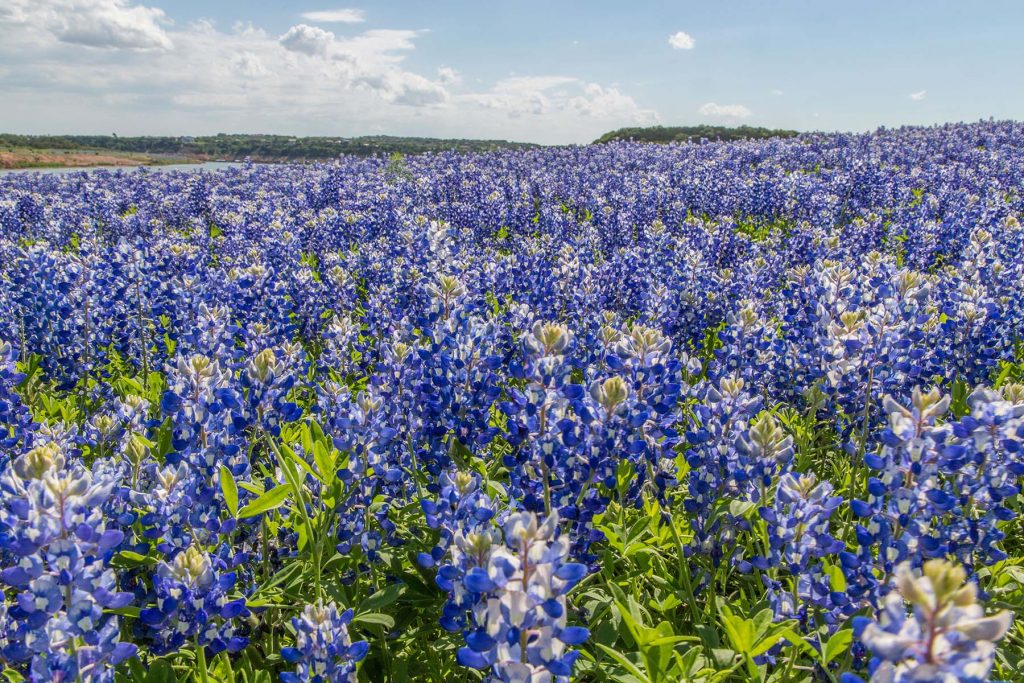The image captures a vast, picturesque field filled with vibrant blue flowers, their hues accentuated with touches of white. Each flower is accompanied by light green leaves and slender stalks. The field stretches across a gently sloping hillside, creating a captivating gradient with the right side slightly elevated compared to the left. In the far distance, a serene horizon of dark green trees forms a natural boundary, beyond which a small lake peeks out from the top left corner. On the horizon, subtle outlines of houses can be seen perched on another hillside. Above, the sky is a crisp blue, adorned with clusters of white clouds predominantly on the left, giving way to a clear expanse on the right. The sunlight bathes the scene in a gentle glow, highlighting the colors and textures, making it a breathtaking portrayal of nature’s beauty.